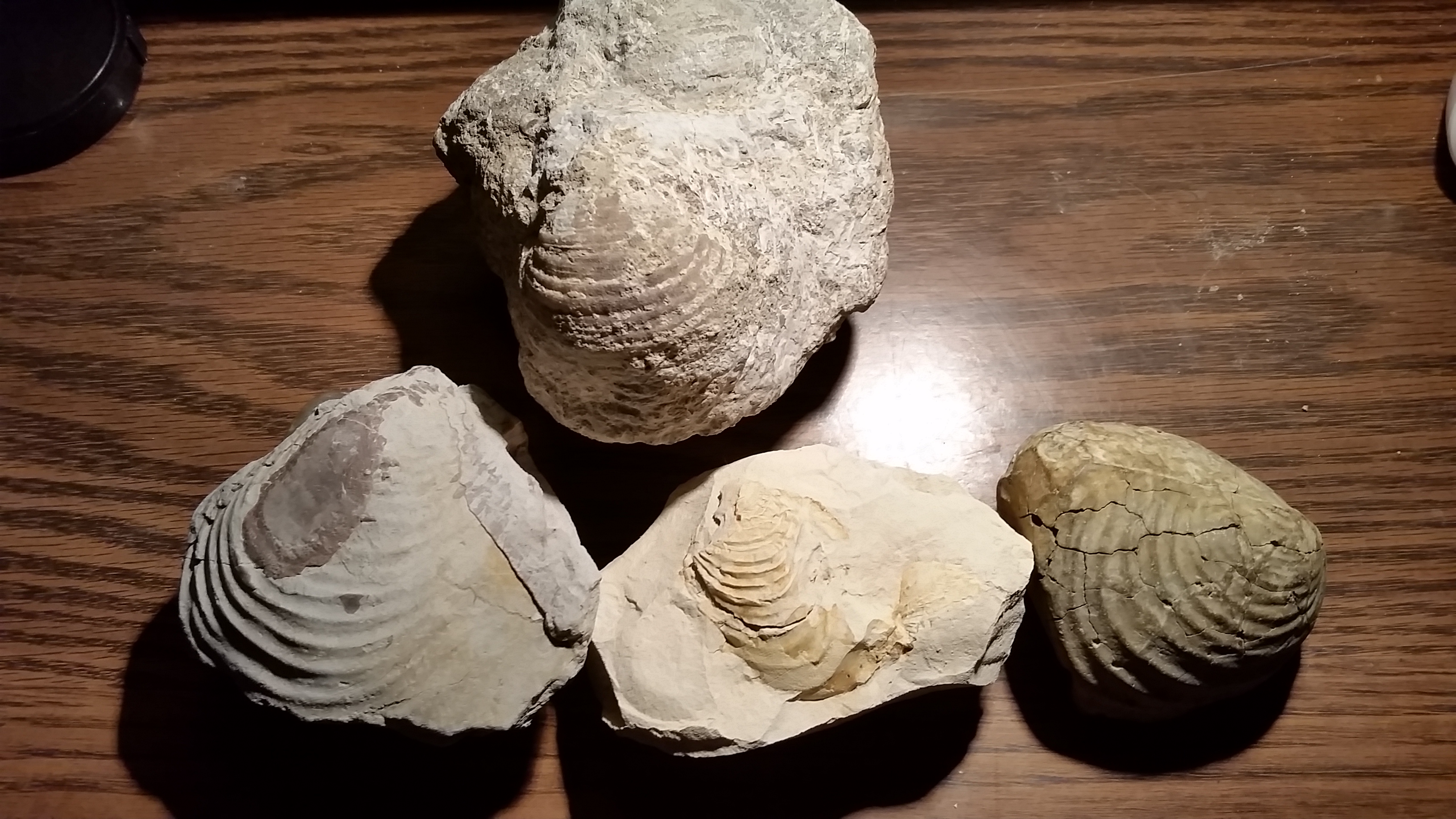This photograph showcases four fossilized seashells arranged on a dark brown stained wooden table, captured indoors with artificial lighting. The image is horizontally rectangular and centers on the shells with a visible reflection from the light source. There are three smaller shells at the bottom and one larger shell at the top, approximately twice the size of the others. The bottom row consists of a gray shell on the far left, an off-white shell in the middle, and a darker, brown shell on the right. The larger top shell is less well-defined, with subdued ridges and a mixed coloration of off-white and brownish tints. These fossils display crevices and a shape reminiscent of crustacean shells such as clams or oysters, having undergone a process where the original calcium material has been replaced by sediment, hardening into rock-like forms.